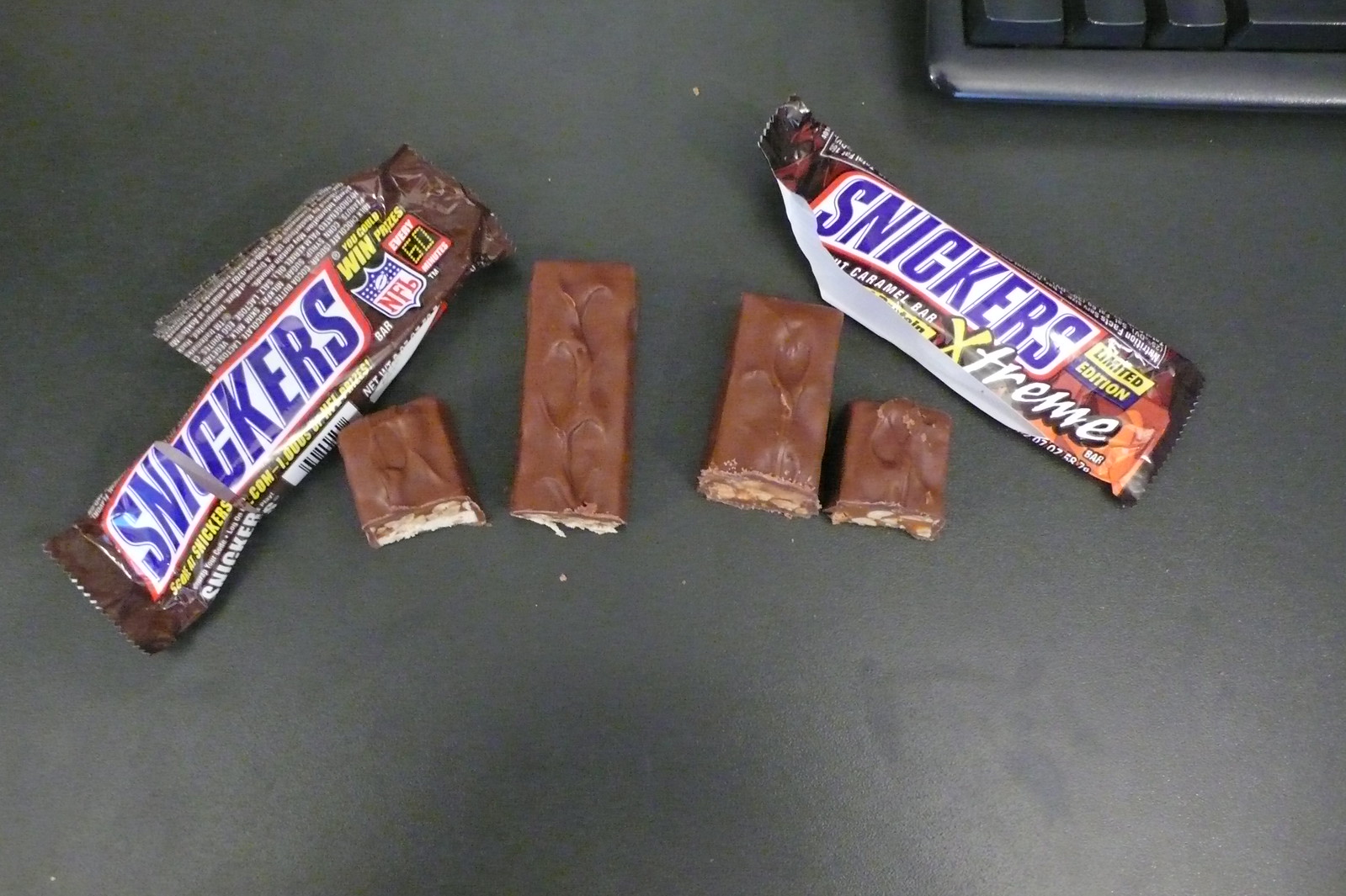The color photograph showcases a dark gray desktop with a partially visible black keyboard in the upper right corner, displaying four keys. Dominating the scene are two Snickers bars and their respective wrappers, arranged diagonally across the surface. On the left, there is a Snickers bar with a wrapper featuring an NFL contest promotion, with its broken candy bar revealing lighter-colored caramel. To the right, the Snickers Limited Edition Extreme bar displays its own wrapper, partially torn but identifiable by the visible "Extreme" label, and features pieces with darker caramel. Both candy bars are divided into two unequal parts, each placed prominently beside their respective wrappers, creating an organized yet casual arrangement.